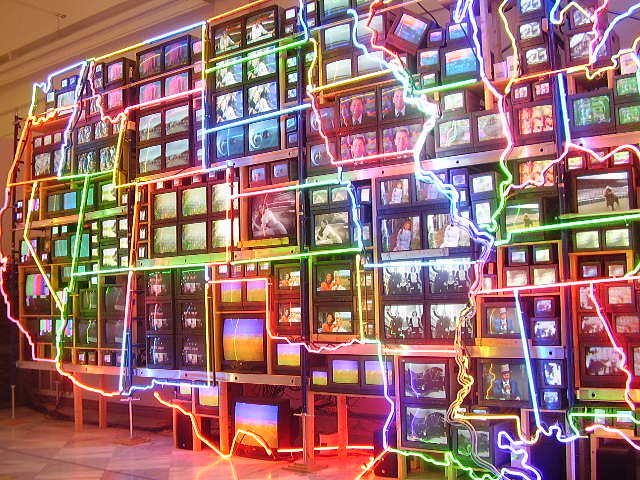This photograph captures an art installation featuring a towering wall of retro-styled television screens, varying in size but predominantly small, arranged to resemble windows or picture frames. The TVs are turned on, each displaying different broadcasts, which collectively appear to represent various U.S. states, with some screens showing content like U.S. presidents and racehorses, suggesting specific states like Kentucky. Overlaying this intricate network of TV screens, all set within a complex shelving system, is an eye-catching neon map of the United States. This neon map is a vibrant tapestry of colors—neon green, orange, red, purple, and white—tracing the state borders from California on the far left to portions of Ohio, Kentucky, Tennessee, and Alabama on the right, with the states on the easternmost side cut off. The neon lights and televised images combine to create a vivid, colorful, and detailed depiction of American geography in this elaborate installation.